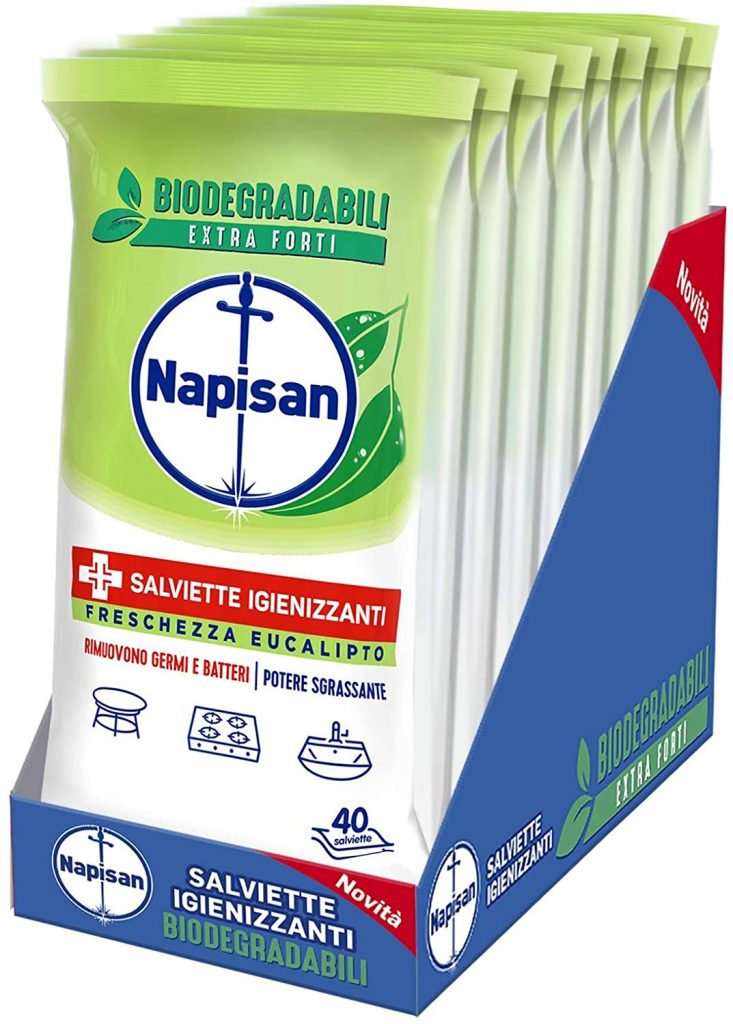The image shows a blue cardboard display containing eight individually wrapped packages of biodegradable wipes. The packaging, predominantly light green and white, prominently features the brand logo “Napisan,” which includes a circle with a downward-pointing sword and green leaves. The central text on the packaging states "biodegradability extra forte" (in Italian), with a horizontal red band that reads "SALVIETTE IGIENIZZANTI, fresca zetta eucalypto" indicating the variety of the wipes and their eucalyptus scent. Additional text on the packaging includes "rimuovono germi e batteri" and "potere sgrassante," highlighting the wipes' effectiveness in killing germs and degreasing. The packaging also includes small blue line illustrations of a table, stovetop, and kitchen sink, indicating the various surfaces the wipes can be used on. The display is angled towards the camera, clearly showing the Napisan logo and design elements on both the front and right side.